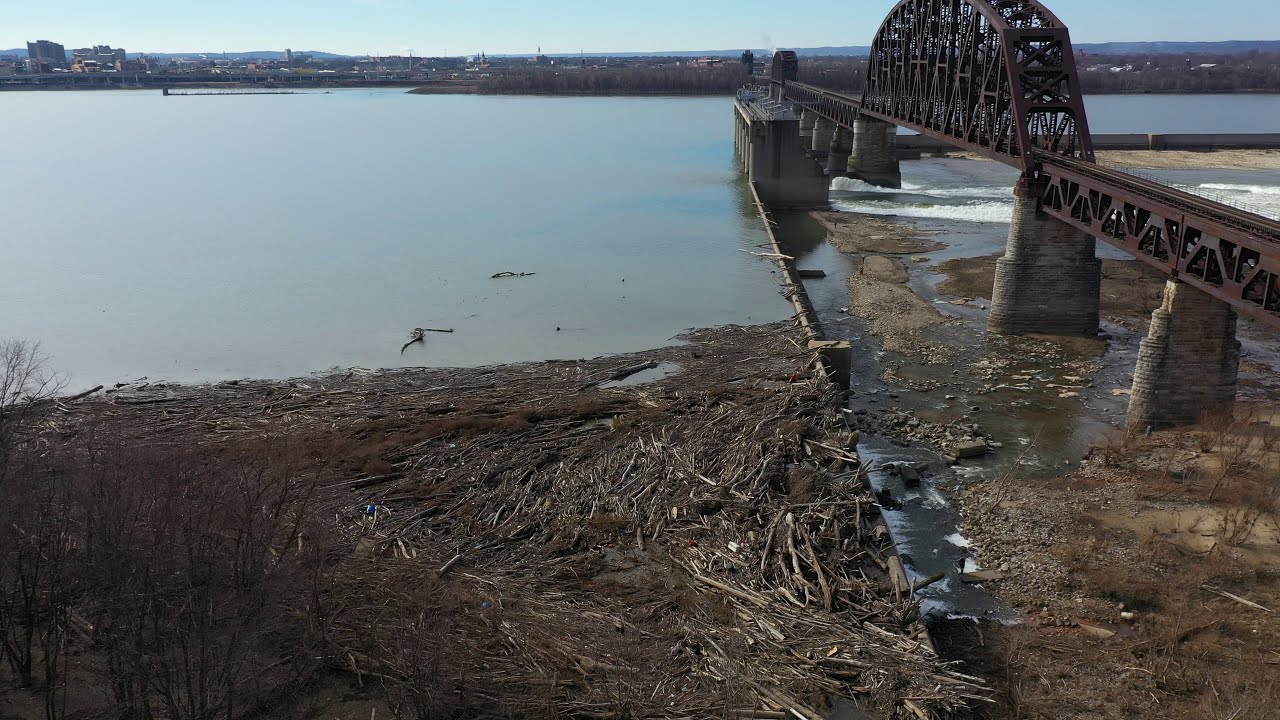The image depicts an outdoor day scene dominated by an old, rusty, dark brown metal railroad bridge with an arch on top, spanning across a shallow and murky river. The bridge consists of at least two arches and extends from the center-right side, slanting upwards towards the top center of the photograph. The bridge supports are made of gray stone or cement. The lower left corner of the image is filled with driftwood and large logs piled against a barrier intended to protect the bridge's pillars. The shoreline, present in the lower part of the image, is cluttered with dry and detached long grass and surrounded by brown, leafless shrubs. In the distance, across the river, there is a glimpse of a small cityscape under a blue sky, accompanied by barren trees contributing to the overall gloomy atmosphere.